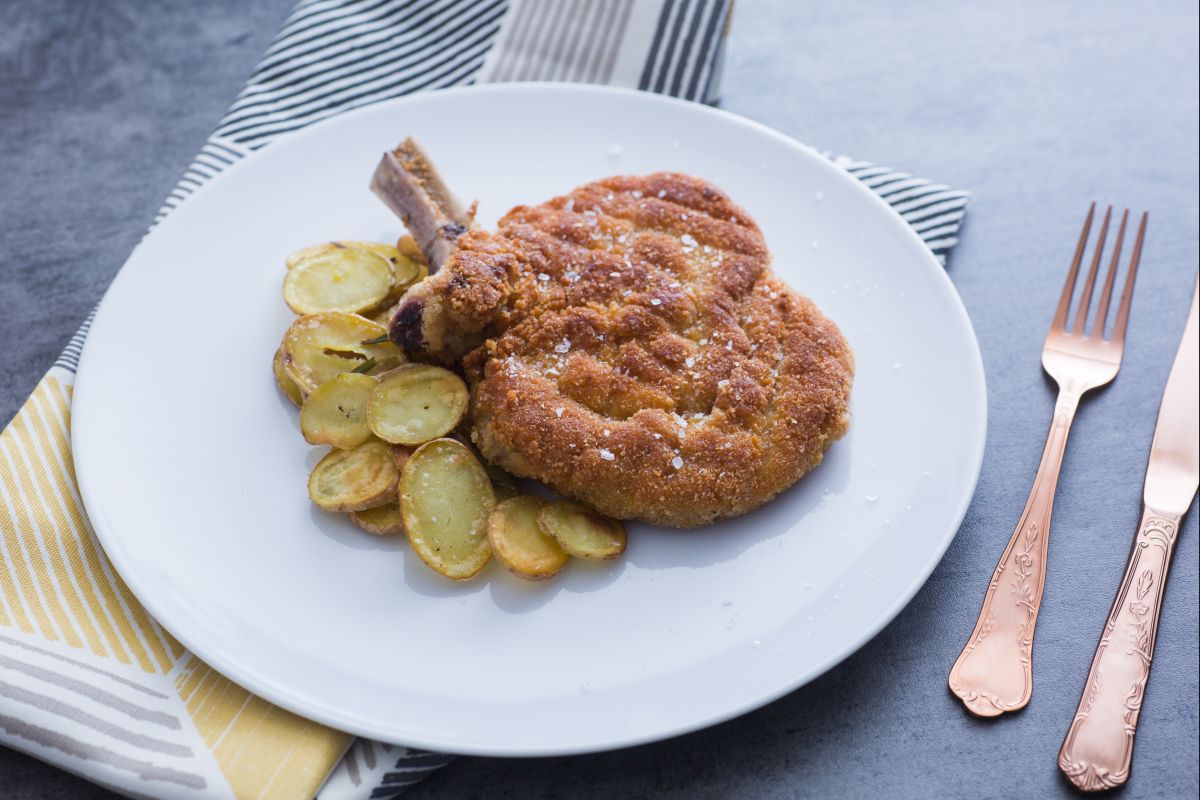This is an overhead photo of a white, round plate of food placed at the center of the image. The plate features two breaded, golden brown pork chops with the characteristic pork chop bone visible on each. Next to the pork chops are crispy, oval-shaped slices of fried potatoes that resemble homemade potato chips. To the right of the plate are two utensils: a fork to the left and a knife to the right, both of which have a shiny, reflective bronze-brown hue with intricate floral swirl designs on their handles. Below the plate, and to the left, lies a napkin with a striped pattern featuring black, gray, and yellow colors. The setup is arranged on a flat, gray surface. The overall composition exudes a sense of elegance and homeliness.